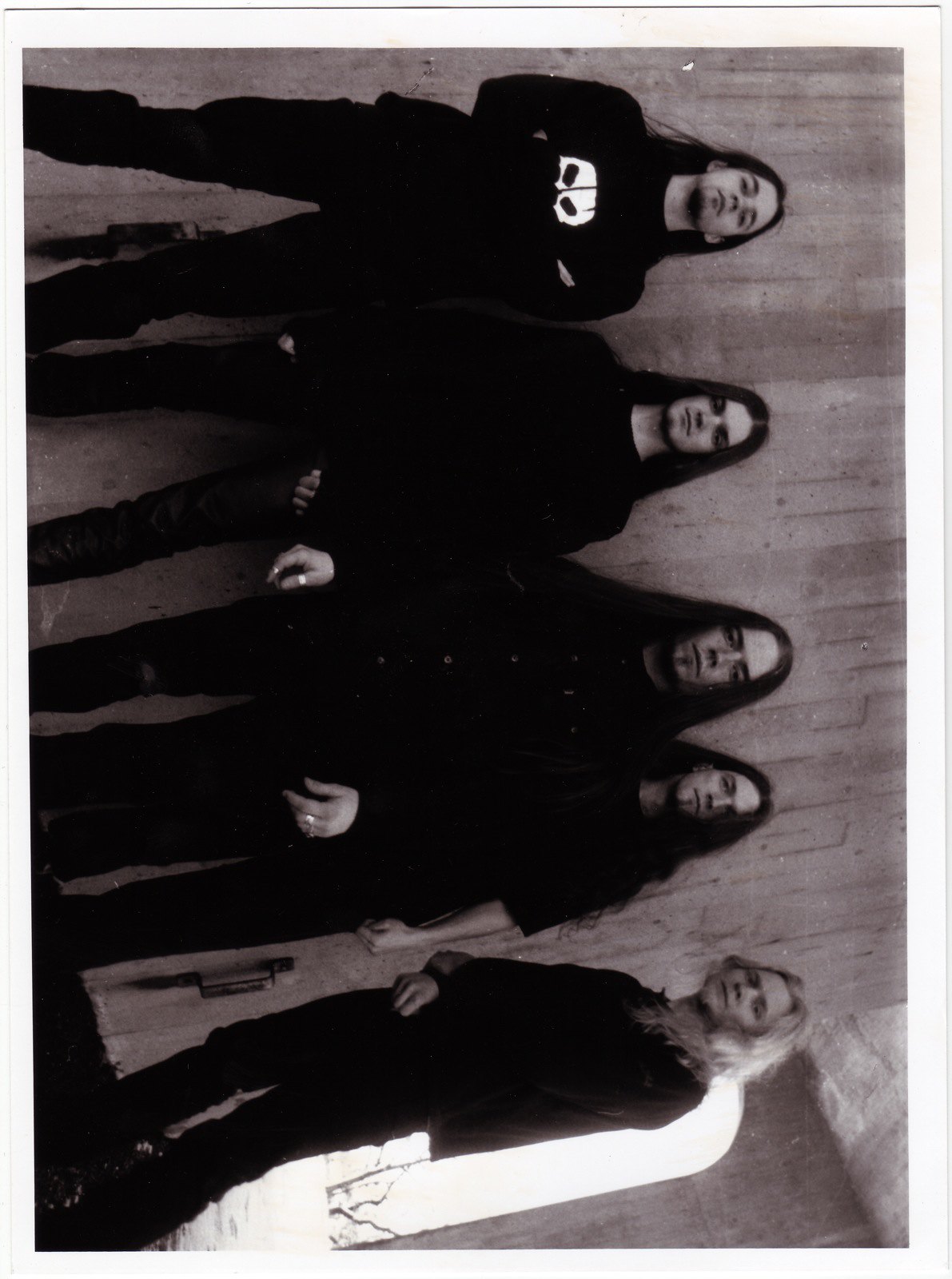The image is an old black-and-white photograph presented with a white border and rotated 90 degrees. It features five men standing against a wall, viewed from left to right. Four of them have long black hair and wear long-sleeve black shirts and black pants; the man on the far left has his arms crossed, revealing part of a white skull image on his shirt. The man to the far right, with long blonde hair, stands slightly turned towards the others. All of them have a somber or neutral expression and several wear rings on their hands. The central figure appears slightly closer to the viewer, and all five men look downward. Behind the blonde-haired man, there’s an archway with light streaming through, suggesting an open pathway. The wall behind them appears stone-like with noticeable striations.